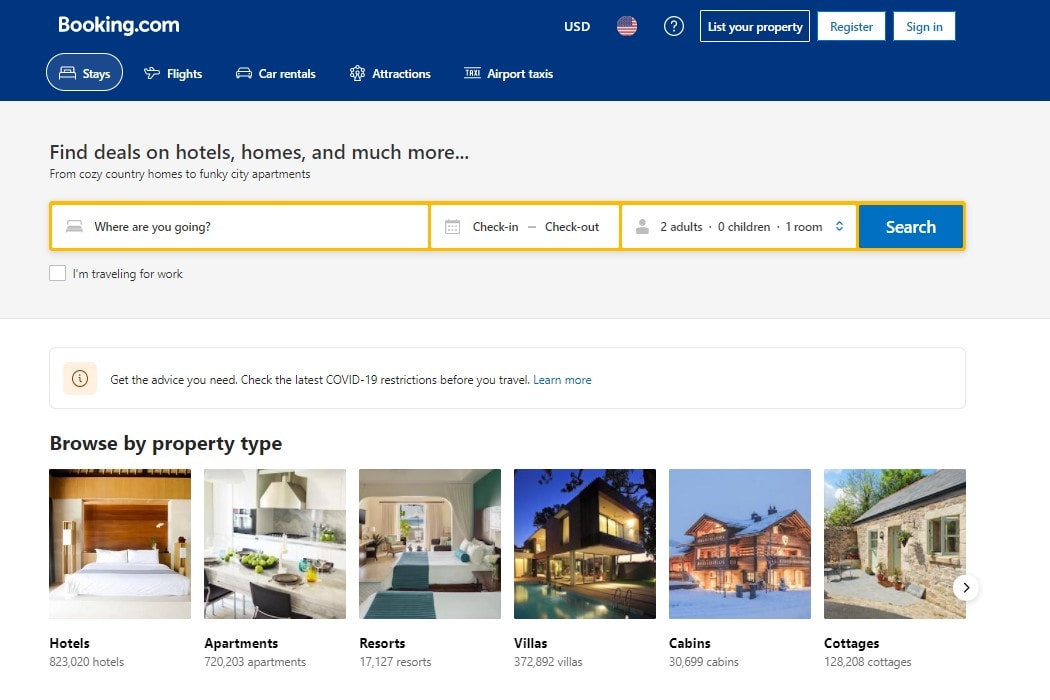In the Booking.com website header, a prominent blue rectangle displays the "Booking.com" logo at the top. On the right side of this blue bar, there are several icons and options: "USD," presumably for U.S. dollars, an American flag, possibly a language selector, a question mark in a circle indicating help, a "List Your Property" button, a "Register" button, and a "Sign In" button.

Below the Booking.com logo on the left, there is a navigation menu featuring options like "Stays," "Flights," "Car Rentals," "Attractions," and "Airport Taxis," each accompanied by an illustrative icon.

Beneath this menu, a gray box invites users to find deals on various accommodations, from cozy country homes to funky city apartments. Directly below, three horizontally aligned text boxes prompt users to enter their destination ("Where are you going?"), check-in and check-out dates, and details about the guest count ("2 adults, 0 children, 1 room"). A prominent "Search" button is situated next to these fields.

Further down, a white rectangle with a gray border contains a clock icon and a message urging users to check the latest COVID-19 restrictions before traveling, with a "Learn more" link.

Finally, the "Browse by Property Type" section showcases six images representing different accommodation categories: hotels, apartments, resorts, villas, cabins, and cottages.